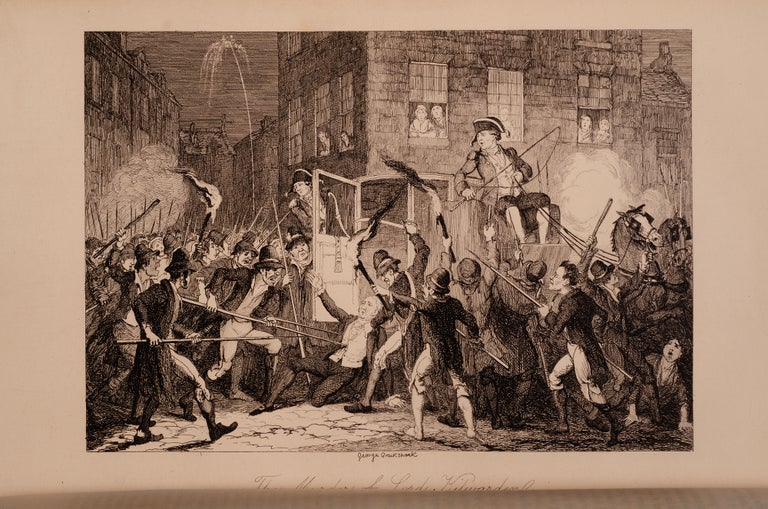The image is a detailed, vintage drawing on aged, beige paper, possibly from the 1700s. The scene depicts a chaotic street battle with old-school buildings framing the background. People peer out from the windows of these buildings, observing the turmoil below. In the foreground, a man is being dragged from a horse-drawn carriage. He lies on the ground as regular townsfolk, armed with guns, spears, bayonets, and pickets, attack him. The men appear as either rioters or protesters clashing with officials, all under the tumultuous presence of smoke, explosions, and fire. The entire scene, rich in detail and drama, is rendered in a manner evocative of historical conflicts, capturing a moment of intense civil unrest. The bottom part of the image contains some obscured writing, likely a signature, adding to its vintage authenticity.